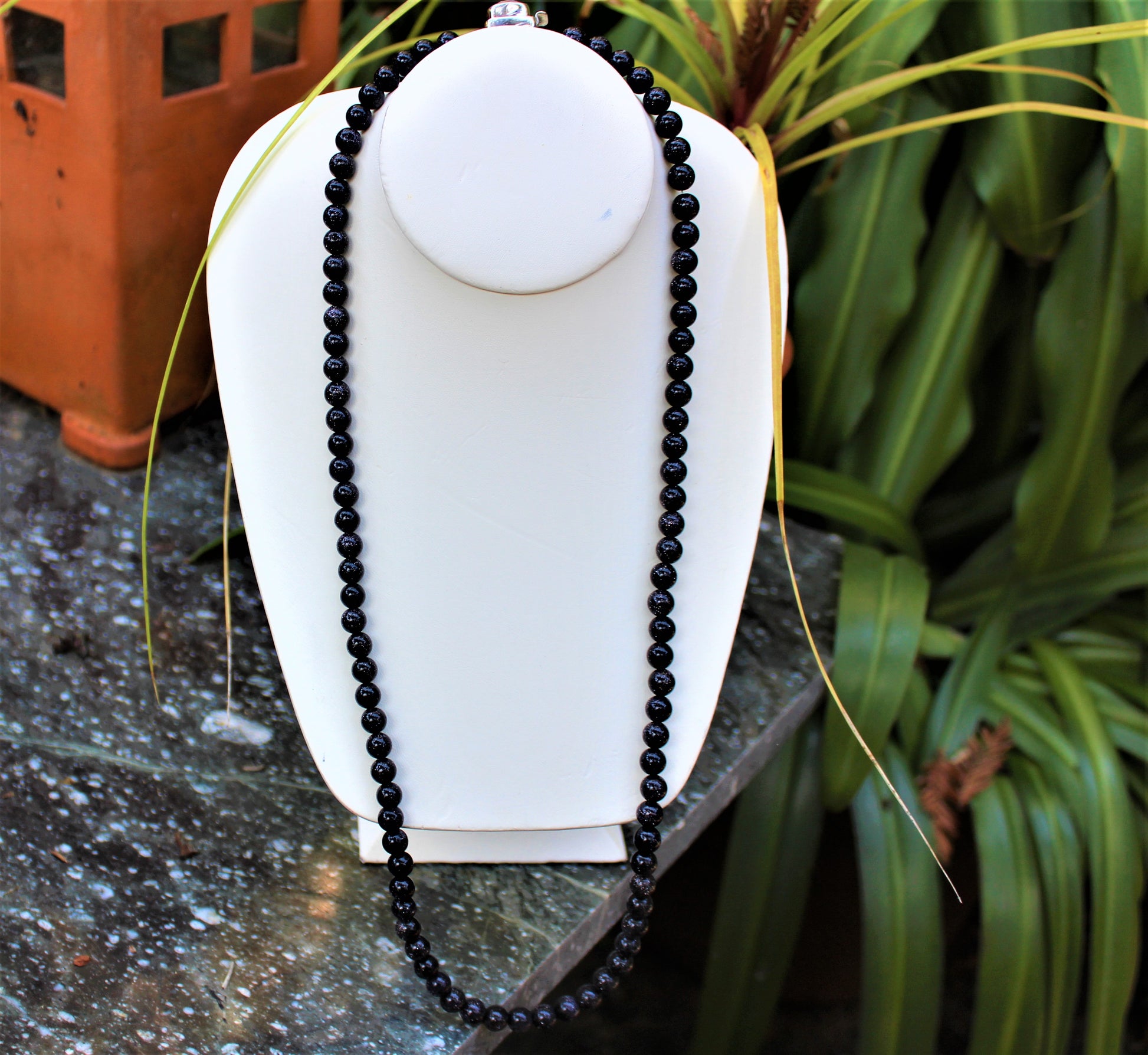This is an outdoor photo featuring a detailed garden setting, centered around a polished, dark-colored granite table speckled with grays. On the table sits a white necklace mannequin form, specifically designed for display purposes, showcasing a lengthy black beaded necklace. The necklace, which likely consists of around 150 beads, possibly black pearls, drapes elegantly from the mannequin's neck down to the table surface. To the right of the mannequin, a spider plant cascades partially over the display form, adding a touch of greenery. Beside the table on the right, a tropical, palmy plant contributes to the lush, garden ambiance. In the top left corner of the photo, a red or burnt-orange box device with small feet and several square openings is partially visible, though some of its details are just out of the frame.